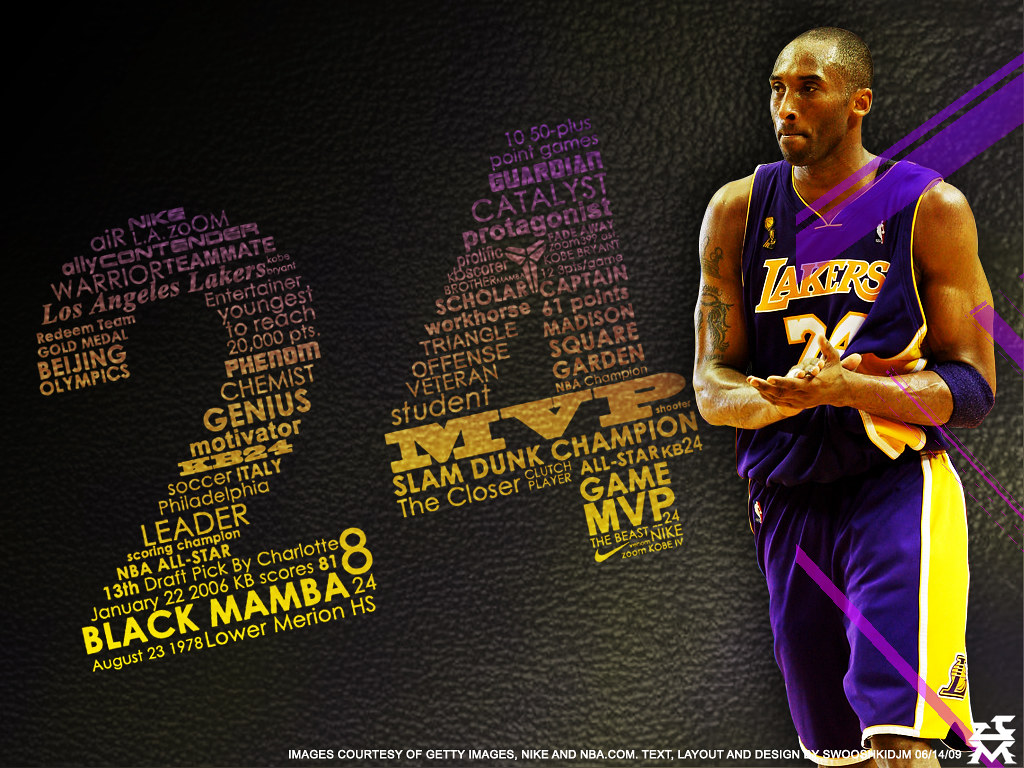The image features Kobe Bryant, a renowned basketball player, standing from the knees up on the right side of the composition. He is an African American male in his mid-30s, attired in a purple and yellow sleeveless Lakers uniform with emblazoned large capital letters "LAKERS" above the number "24" on his chest. His left forearm bears a tattoo, while his right arm is adorned with a purple band. Kobe stands with his arms crossed, facing towards the left, not directly looking at the camera.

The background is a textured gradient that shifts from charcoal to light gray, interspersed with black elements. On the left side of the image, a large number "24," fading from purple at the top to yellow at the bottom, occupies about 40% of the background. This number "24" is composed of various inspiring words and phrases associated with Kobe Bryant, such as "slam dunk," "champion," "Black Mamba," "leader," "genius," "phenom," "MVP," "game MVP," "chemist," "Beijing," and "Olympics." The overall feel is digitally created, emphasizing a heroic and commemorative atmosphere through its vivid color scheme including shades of purple, yellow, white, black, and light purple.